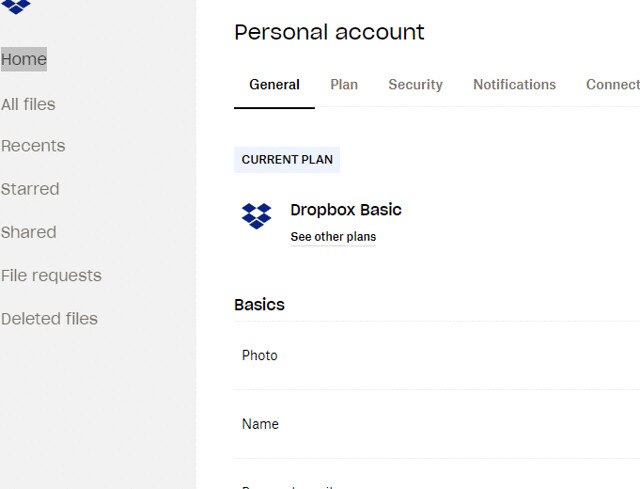This image is a screenshot from a computer interface featuring a prominently white background, complemented by a vertical grey navigation bar on the left. At the very top of the grey bar, in the top-left corner, there are three small triangles arranged in a triangular formation. Below this, a list of menu items appears, each on its own row: "Home," "All Files," "Recent," "Start," "Shared," "File Request," and "Deleted Files," each separated by distinct rows that presumably act as dividers.

In the primary white section of the screenshot, the top segment displays the title "Personal Account." Beneath this designation lies a navigation row with tabs labeled "General," "Plan," "Security," "Notification," and "Connect," each separated by small spaces. The next row features a light blue rectangle labeled "Current Plan."

Further down, there is a cluster of blue triangles similar to those seen in the grey bar, now enriched with two additional triangles sitting atop the original group. Adjacent to this cluster, the text "Dropbox Basics" is visible. A prompt, "See Other Plans," appears directly below this.

Another section follows, starting with the larger-font text "Basics." Below this, the terms "Photo" and "Name" are aligned vertically, each followed by grey horizontal stripes stretching across the entire screen width. The very bottom part of the screenshot is partially obscured, only allowing the top of the letters from an unreadable text to be seen.